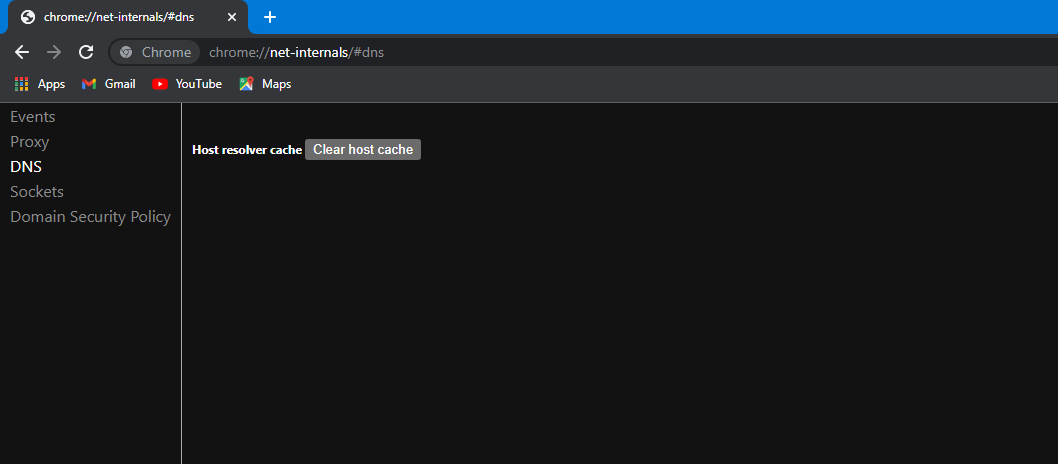The image predominantly features a dark interface, with the majority of the background rendered in black. At the top of the image, a narrow blue bar is visible, followed by a black internet browser tab displaying an address bar with text in white and light gray. The tab includes a small white 'X' for closing the tab. 

To the left of the address bar, there is a back arrow, a forward arrow, and a refresh button. On the left side of the tab, there's a red square with a white triangle, signifying the YouTube logo, and the word "YouTube" written next to it in white. Adjacent to the YouTube icon is another square featuring a combination of green, blue, white, and yellow colors arranged to resemble roads, representing the Google Maps logo, with the word "Maps" written next to it in white.

Centered on the black background, the words "Host Resolver Cache" are displayed in white, alongside a light gray box that reads "Clear Host Cache" in white text. On the left margin of the image, there are several terms written in gray: "Events," "Proxy," "DNS," "Sockets," and "Domain Security Policy." Additionally, the word "Gmail" appears in white text as part of the interface. Overall, the image captures a detailed view of a browser UI with emphasis on navigation and application icons within a predominantly dark theme.